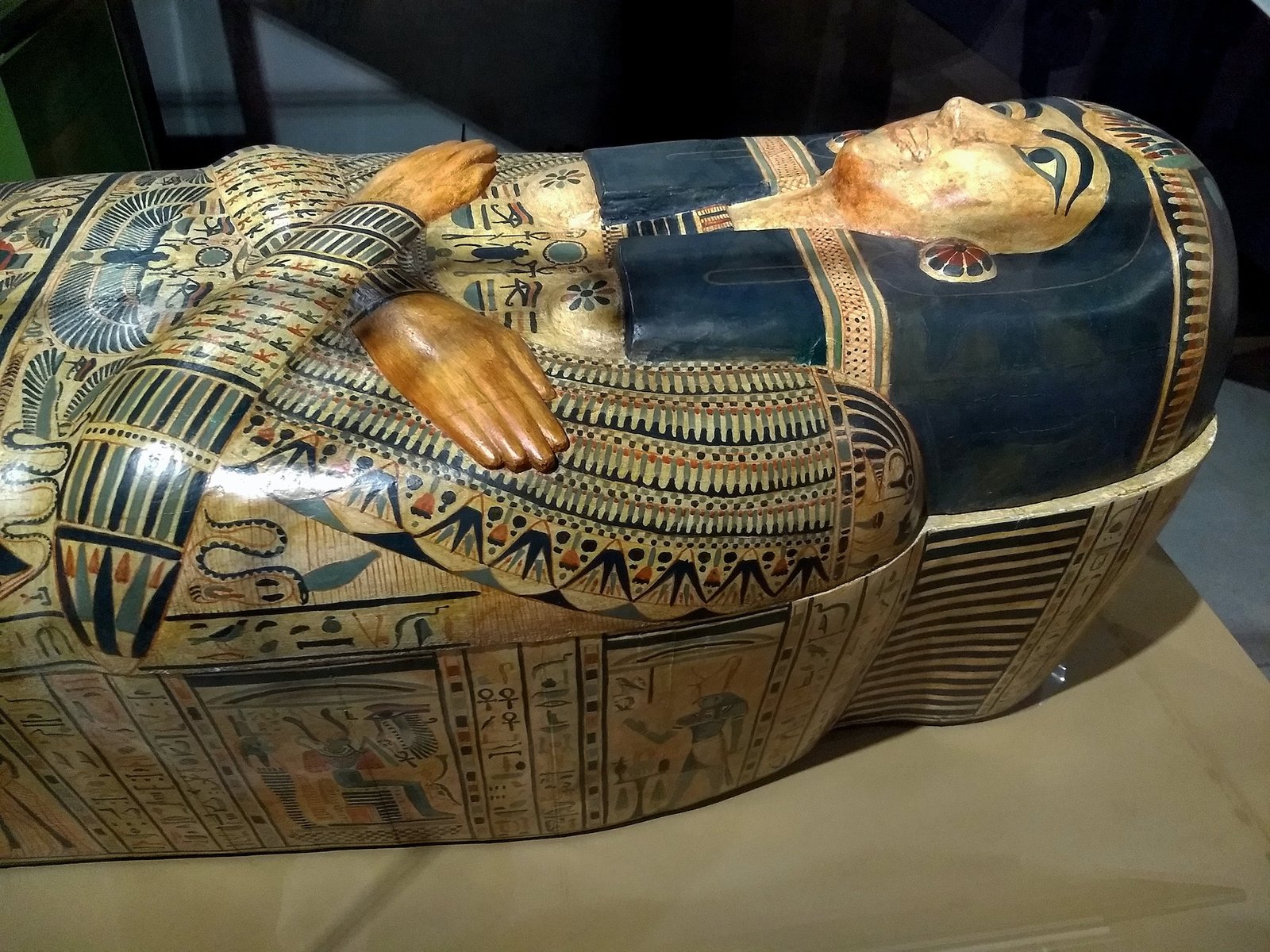The photograph displays a detailed side view of an ancient Egyptian sarcophagus, reminiscent of a pharaoh's casket. The depicted casket lays on a brown paper ground, emphasizing its rectangular shape, which is wider than it is tall. The sarcophagus appears to be in good condition, with intricate Egyptian hieroglyphics and scenes painted all over it. A distinctive carved face, bearing a resemblance to Cleopatra or a pharaoh, crowns the top of the sarcophagus, adorned with thick dark eyebrows and lined eyes. Below the face, the figure's carved arms and hands are crossing over its chest, typical of Egyptian burial customs. Surrounding the chest, and extending downwards, is a painting of a phoenix in brown hues. The predominant colors on the sarcophagus include deep greens, golds, oranges, and blacks on the wood carving. The background of the image is a contrasting dark blue-black, which enhances the intricate, cream-colored designs and details on the casket's upper portion. Detailed engravings of hieroglyphics and other Egyptian motifs cover its entire surface, adding to the rich, historical texture of the artifact.